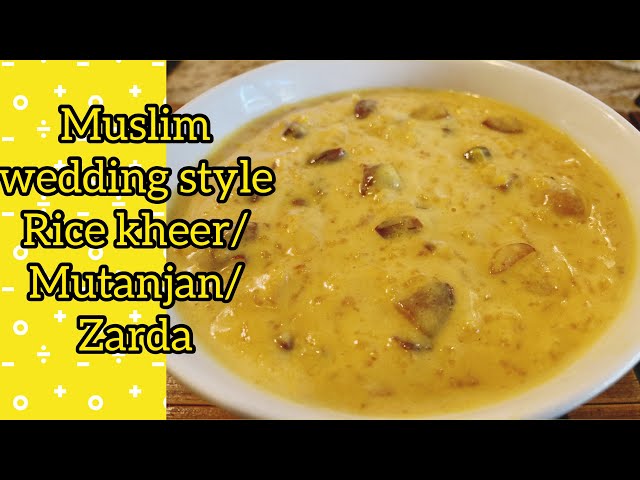This image is a close-up thumbnail likely meant for a YouTube video or a cooking guide, prominently featuring a dish described as "Muslim Wedding Style Rice Kheer / Mutajan / Zarda." The background of the thumbnail includes a yellow design with floating plus and minus signs and circles, covering about a sixth of the screen. The bowl of food, positioned on a medium brown wooden slatted table, contains a yellowish, creamy mixture that resembles a soup or rice pudding, with chunks of potato or possibly sausage. The text, written in yellow font, appears partially on the yellow background and partially over the bowl of food, indicating the celebratory nature of this rich, cheese-like rice dish.